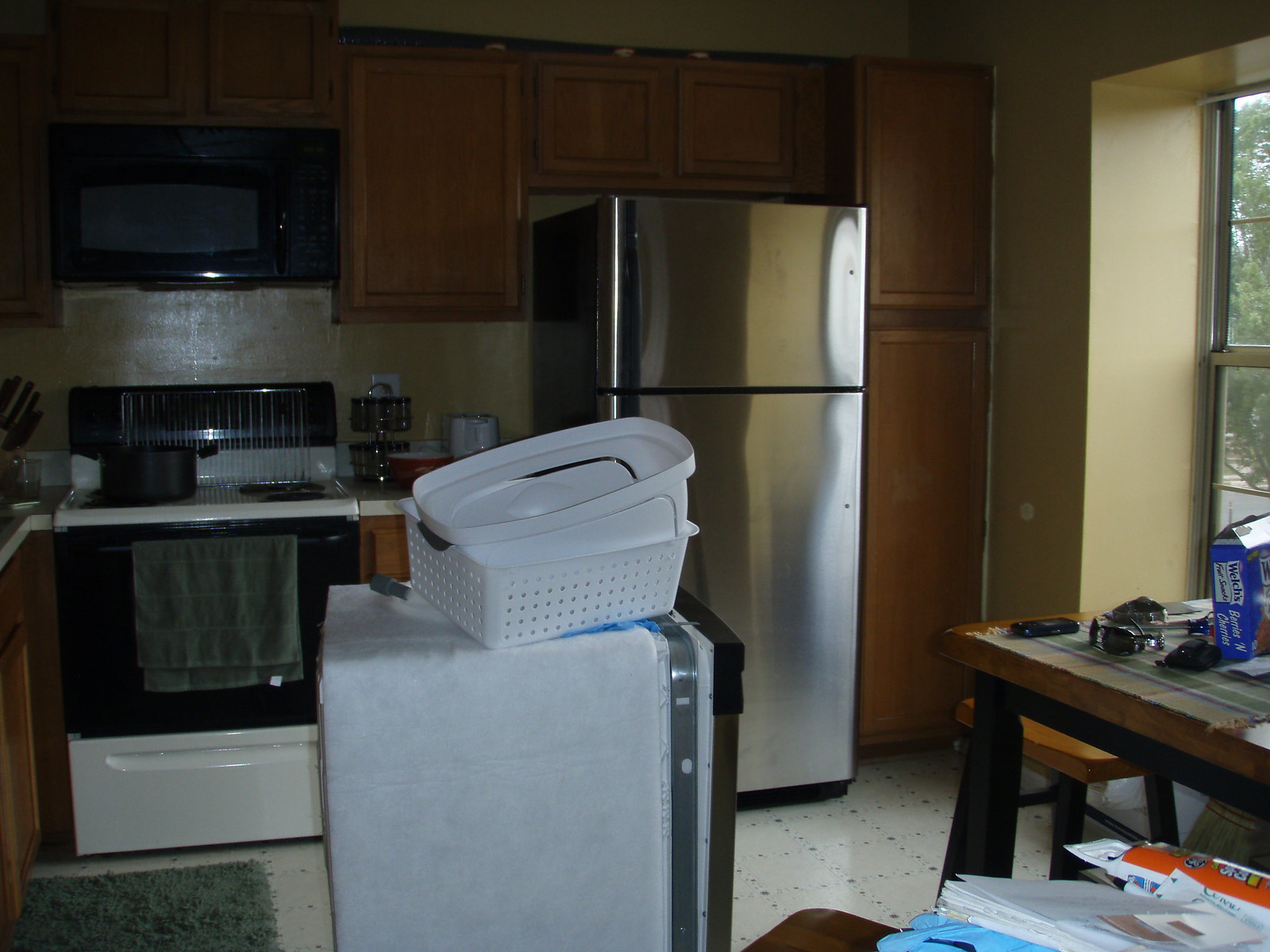The photograph showcases a well-used kitchen, likely captured with a digital camera given the image's coloring. Central to the scene is a large silver refrigerator with a dual-compartment design: the bottom section functioning as the fridge and the top as the freezer. To the left of the fridge, there's a stove and oven combination, with a pull-out tray beneath presumably for storing pans. Above the stove, several wooden cupboards align the top of the area, and a black microwave sits conveniently on top of the stove.

On the right side of the image, we observe a dining table set with placemats. The table contains a box of Welch’s Fruit Snacks in the berries and cherries flavor, a phone, a pair of glasses, and what appears to be a wallet. Closer to the camera on the same table is a stack of mail alongside a can whose label is not legible due to its angle.

Dominating the middle of the kitchen area is an appliance, likely a dishwasher, that has been pulled out from its usual installed position, indicating some form of maintenance or installation in progress. The overall setup and visible items hint at a busy household in the midst of daily life.